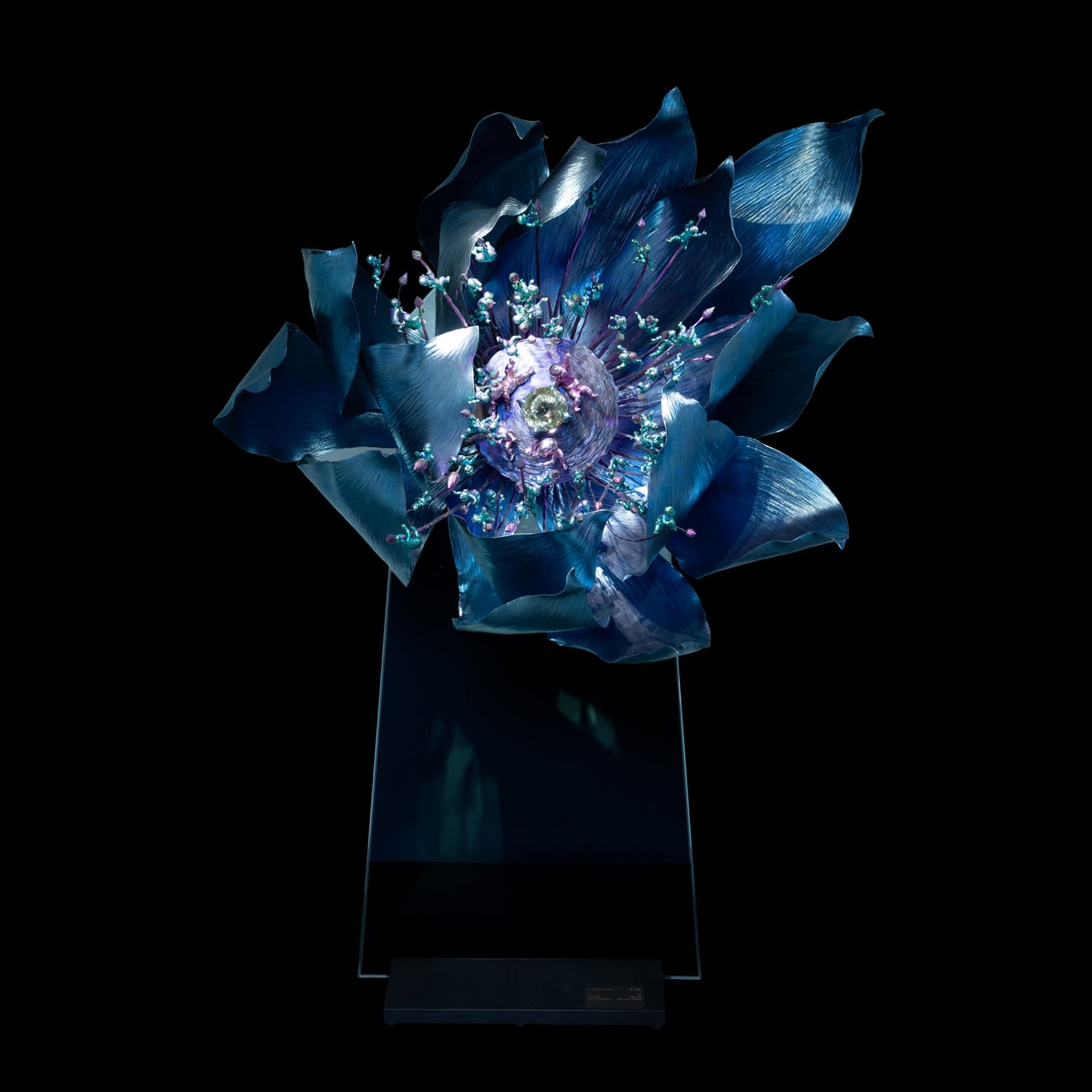This striking and futuristic sculpture, set against a solid black background, showcases an intricate flower design atop a sleek, matte black podium. Illuminated from above, the sculpture captures attention with its dynamic sense of movement. Bluish-green petals, some elegantly bent and curved, extend from a central purple bud, adorned with sprouting yellow and light blue spiky elements reminiscent of pollen. The flower stands at the top of a glass sheet, approximately 3 feet wide and 4 feet high, which is slotted into the base. Adding to its intriguing composition, the sculpture appears to be crafted from a stiff, possibly metallic material that is blue and black. The base features a discreet plaque, although the inscription isn't legible, further enhancing the mystery and allure of this captivating art piece.